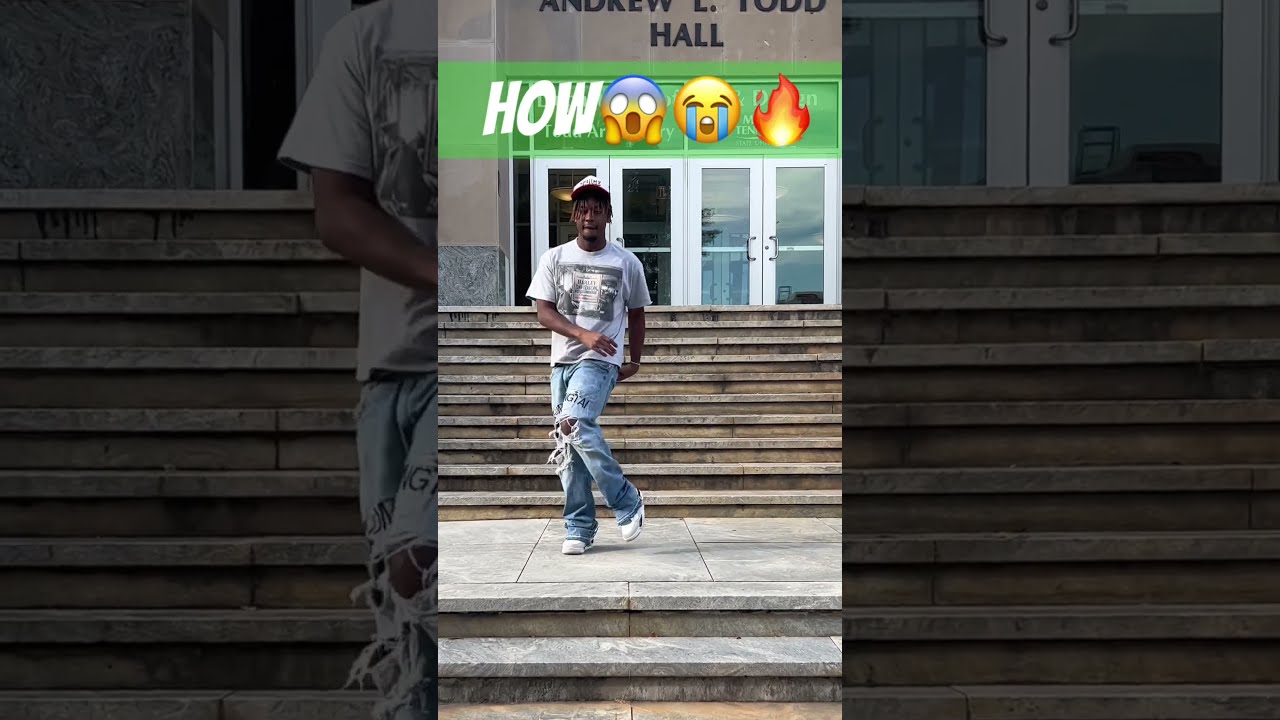The photograph captures a young African American male with medium-length, chin-reaching dreadlocks poking out from under a white baseball cap with a red brim. He appears to be dancing on a small platform flanked by two sets of gray cement steps outside a building identified as Andrew E. Todd Hall. This hall entrance features four glass doors, above which the building's name is clearly displayed. The man is clad in a gray short-sleeved t-shirt adorned with a black-and-white logo, light blue distressed jeans featuring prominent holes at the knees, and white sneakers. His animated pose suggests he's either performing a dance move for a TikTok video or some similar social media content, as his right hand is extended in front, and his left hand appears to be positioned behind him with his left leg curving forward. Above him, there's a green banner with "HOW" inscribed in white capital letters and a sequence of three emojis: a shocked face, a crying face, and a flame. The surroundings, coupled with his outfit and dynamic stance, vividly portray the expressive moment amid a collegiate environment.